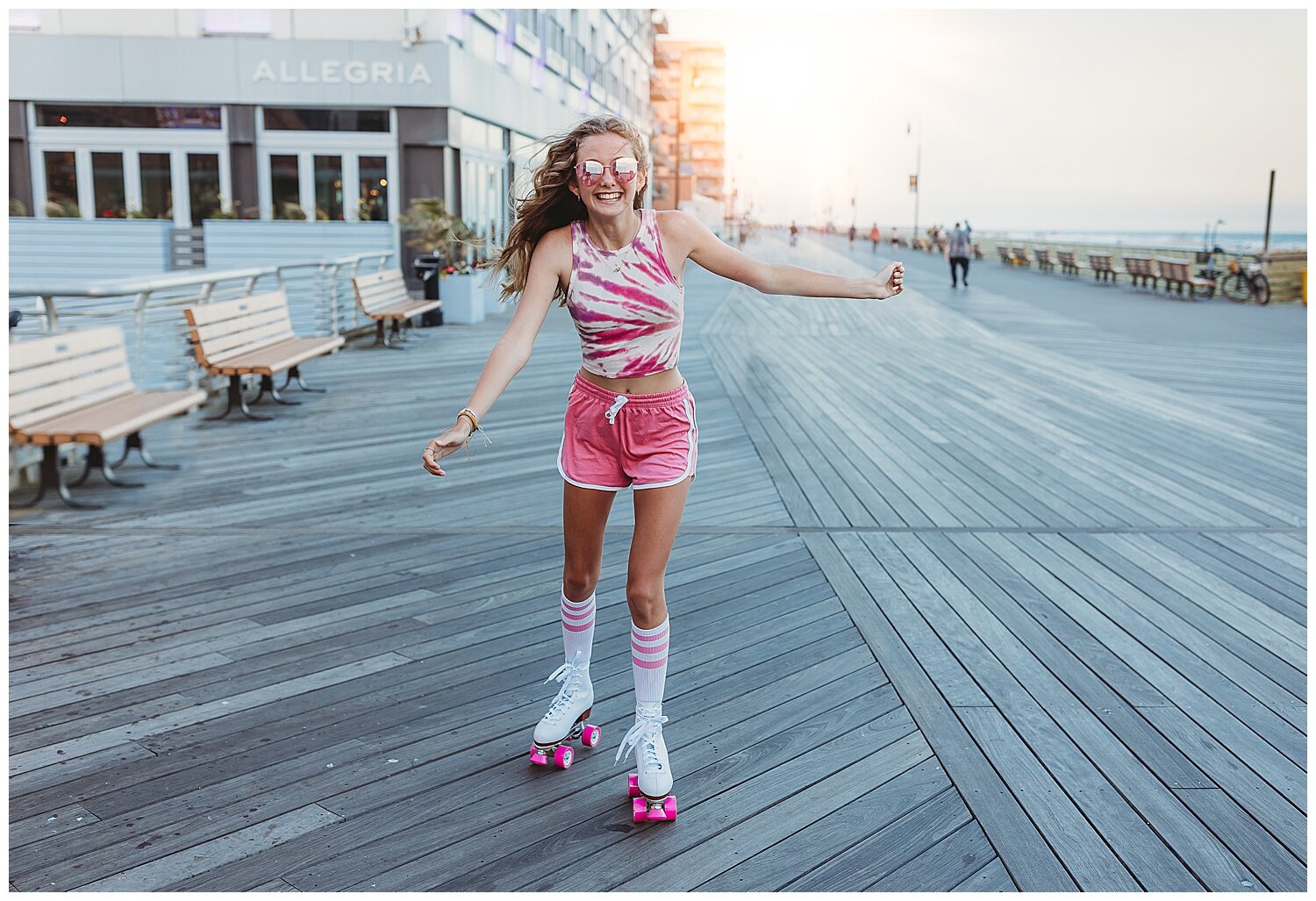The photograph captures a vibrant scene of a young woman, who appears to be in her early 20s, roller skating along a well-maintained, gray wooden boardwalk by the ocean. Her light brown, wavy hair flows halfway down her back, complementing her playful attire that includes amber-colored round sunglasses, a pink and white tie-dyed tank top, and matching pink jogging shorts with three white stripes on the sides. She sports white knee-high socks with pink stripes at the top and white roller skates equipped with bright pink wheels. The woman smiles directly into the camera, exuding joy and energy under the midday sun. To her left, a series of wooden benches line the boardwalk, while a tall, multi-story building stands in the upper left corner of the scene. In the upper right, the sparkling ocean and sky are visible, adding to the picturesque coastal setting. Additionally, another beige building and several additional benches, along with a few pedestrians, can be spotted in the background, contributing to the lively ambiance of the boardwalk.